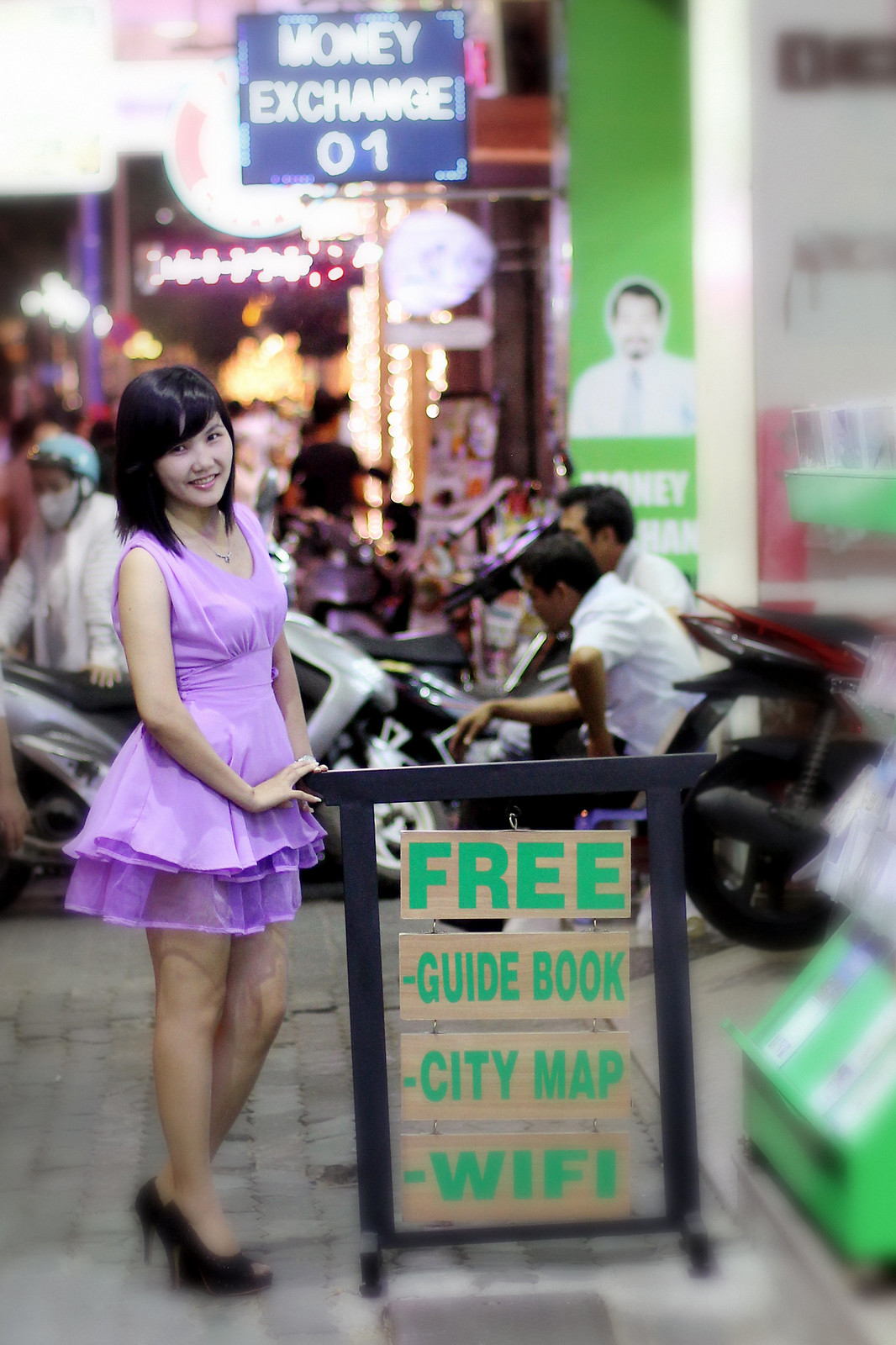The photograph captures a bustling city street, likely in an Asian metropolis, with a young Asian woman as the focal point. She has medium-length black hair and is wearing a sleeveless purple dress with a short skirt, paired with high black heels. She is standing next to a black rectangular street sign post, which appears to be a movable promotional stand. The sign features brown wooden panels with green lettering that reads: "Free guidebook, city map, Wi-Fi." The woman smiles directly at the camera, her hand resting on the sign post. 

In the background, the street is lively with multiple people visible, including several men seated on a stoop beside parked motorcycles. One man on the left wears a face mask and a blue motorcycle helmet. The backdrop is illuminated with various business signs and bright lights, contributing to the busy atmosphere; one prominent sign is blue with white lettering that reads "Money Exchange." The scene around the woman is slightly blurred, emphasizing her as the main subject against the dynamic cityscape.